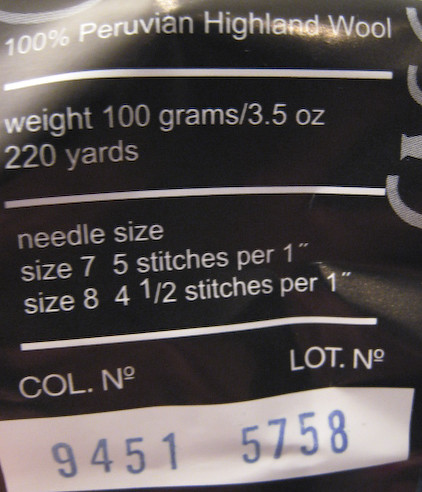In this image, a detailed label with a slightly wrinkled black background appears to be affixed to a bag or packaging. The label prominently features knitting details. At the top, "100% Peruvian Highland Wool" is clearly printed, indicating the material. Below, a white line separates this header from the following specifications. 

Detailed knitting needle sizes and stitch counts are listed: 
- Size 7 needles yield 5 stitches per inch.
- Size 8 needles yield 4.5 stitches per inch.

Further down, the label specifies the weight and length of the wool: "100 grams, 3.5 ounces, 220 yards." The repeated information about needle sizes appears once more for emphasis. 

Additionally, the label includes a color identifier "COL" followed by a dot and a specific number, as well as a lot number stated below. The numbers "9451" and "5758" are legible. Some indistinct writing is present on the side of the label, but it is too unclear to be deciphered.